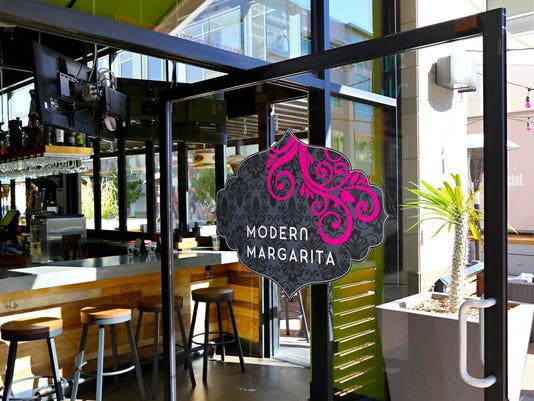The photograph captures a sleek, modern restaurant named "Modern Margarita," characterized by its extensive glass architecture. At the forefront of the image, a circular sign resembling a balloon prominently displays the restaurant's name in large white letters, accompanied by bright pink swirls and floral patterns. The entrance door is open, revealing an inviting interior. Immediately inside, there is a white planter with a small palm tree adding a touch of greenery. Through the expansive glass walls, the contemporary design is evident with black metal frames supporting the structure. Inside, wooden bar counters and stools with brown seats and grey metal legs create a warm ambiance. Glasses are suspended above the bar area, which also features a white countertop and a visible cash register. Televisions mounted above the bar further emphasize the modern atmosphere. The setting appears inviting yet devoid of patrons, highlighting the open, spacious layout with clear views through the glass to another similarly modern building in the background.